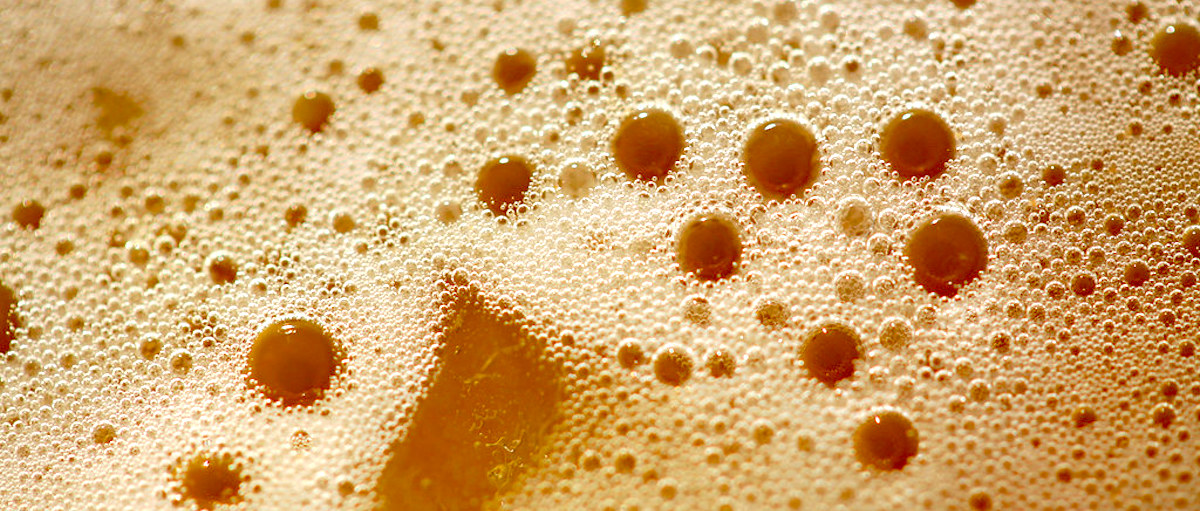The image depicts a very close-up view of a liquid surface filled with bubbles. The liquid appears to be a deep amber-yellow, resembling the color of tea or a lightly poured beer, with hints of orange and brown. The bubbles vary in size, creating a textured, foamy appearance. Tiny bubbles spread across the entire surface look like a fine white foam, while larger bubbles stand out more prominently. The arrangement of larger bubbles forms distinct clusters, especially noticeable at the center and towards the left side of the image. The overall composition evokes the look of a freshly poured amber-colored beverage, covered in frothy bubbles.